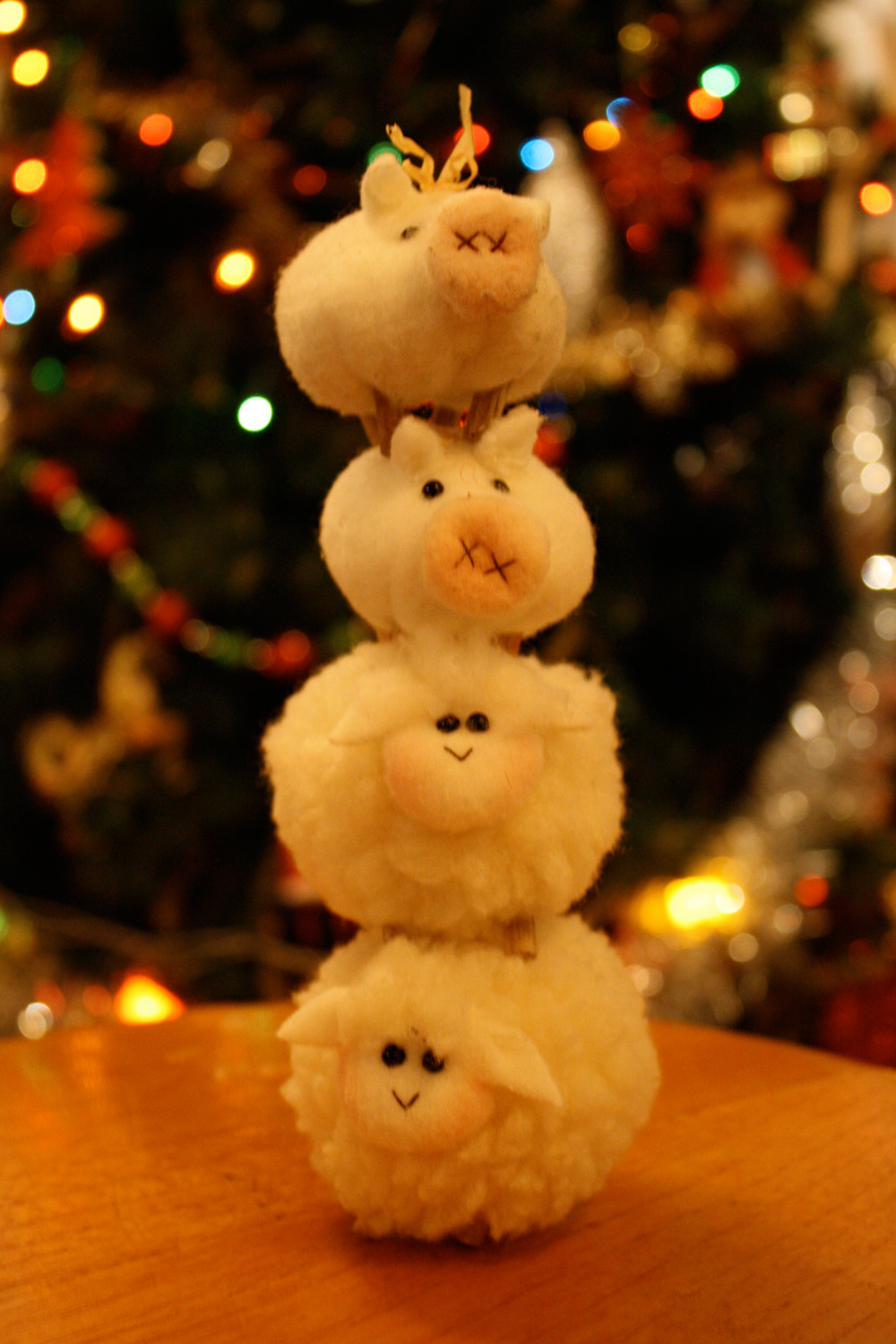In this vertical image, a quartet of small, handmade plush animals are carefully stacked atop a light brown wooden table. At the bottom of the stack are two fluffy lambs with solid white fur, round black bead eyes, and V-shaped red smiles. Above them sit two pigs, slightly smaller, with soft, light pink bodies, large circular snouts adorned with black X's for nostrils, and matching black eyes. Their legs are rendered in brown, possibly wooden material. The whole arrangement is likely held together by a rod for stability.

The background reveals a blurred-out Christmas tree adorned with silver garlands and strands of red, green, and white beads. Additional decorations appear indistinct, adding to the festive atmosphere. Interspersed among the ornaments are glowing blue, yellow, and red lights, contributing soft flares to the scene. The ambient, warm interior lighting casts an orangish hue on the otherwise white and light pink animals, imbuing the scene with a cozy, holiday glow.